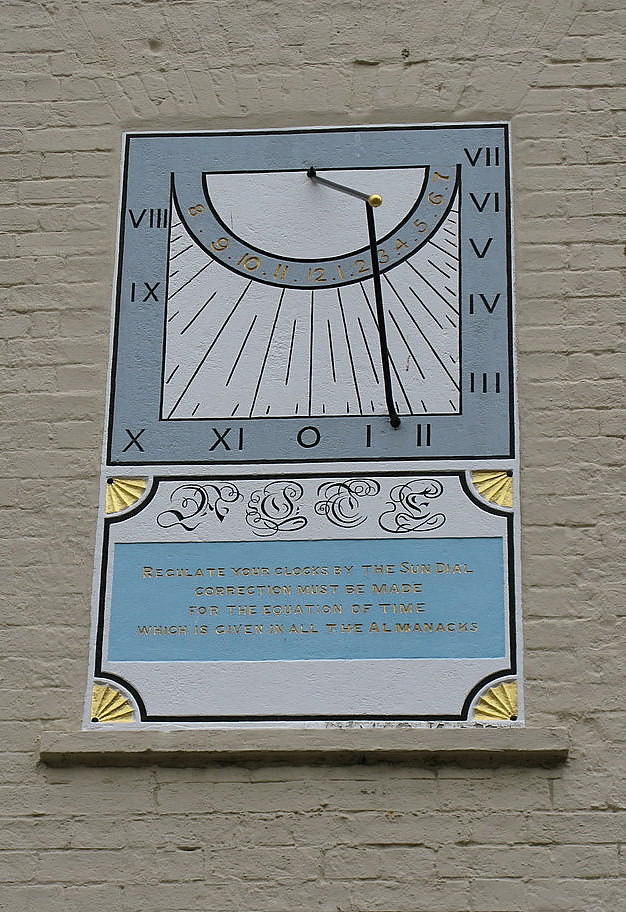The image depicts an antique-style sundial mounted on a white-painted brick wall. The sundial's face is divided into two main sections. The upper portion consists of a gray square featuring a semicircle at the top with radiating lines, designed to utilize the sun for timekeeping. Below the semicircle, there is a misaligned arrangement of roman numerals from 1 to 12, giving it an abstract appearance.

The lower portion of the sundial is a white rectangle that houses a smaller blue rectangle containing gold text. The inscription reads: "Regulate your clocks by the sundial. Correction must be made for the equation of time which is given in all of the almanacs." Each corner of this rectangular section is adorned with yellow fan-like decorations.

The entire piece is fixed against a backdrop of white bricks, lending a classic and historical ambiance to the setting. At the base of the artwork, there is a ledge made of brick, further emphasizing its architectural placement on the building.